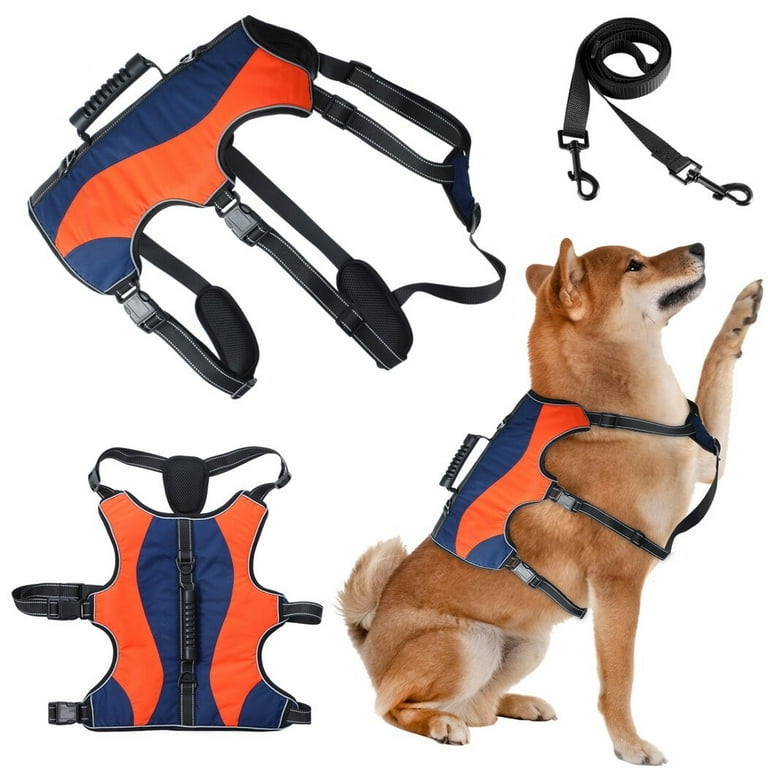The image is a detailed advertisement for a dog harness, featuring a brown and white Shiba Inu sitting and facing the right. The dog, with its curled tail and cream-colored underbelly, wears a blue and orange harness with distinct black straps. These straps include one under the belly, one in front of the front legs, and one around the lower neck, featuring a handle on the back for easy control. The main photo shows the dog with its left paw raised and right paw grounded. Complementary images around showcase different perspectives of the harness: a top-down view in the lower left, a side view in the upper left, and a coiled black leash with two clips in the upper right, all set against a plain white background.